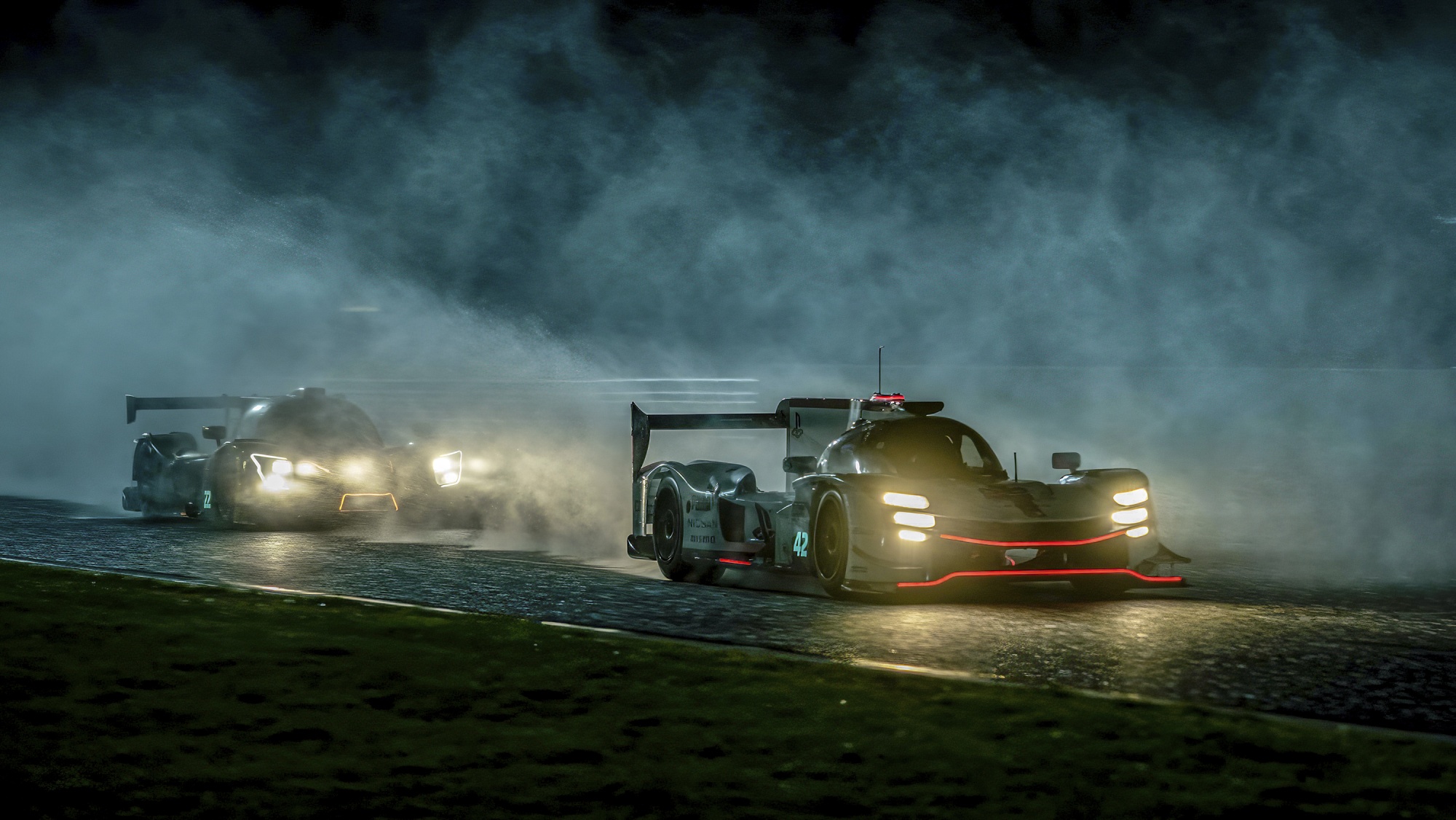In the image, taken at night, two drag race cars dominate the scene, their forms partially obscured by swirling clouds of steam or smoke rising from the road or racetrack. Both vehicles feature rear spoilers and sit low to the ground, indicative of their racing design aimed at reducing wind resistance. The car in the foreground is predominantly white with distinctive red trim along several edges, while the more blurred car in the background appears white as well, with a noticeable yellow trim possibly outlining a license plate area. The hazy atmosphere, filled with dense fog or smoke, suggests a high-speed event or perhaps a loss of control further amplifying the dramatic effect with shadowy silhouettes and diffused light. Despite their potentially flimsy appearance, these cars are built to be as safe and powerful as any standard vehicle.